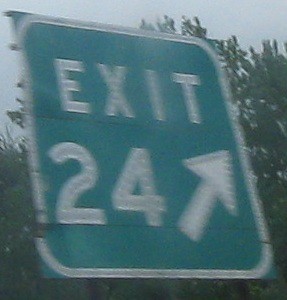This image captures a slightly blurry and pixelated highway exit sign against a backdrop of tall, leafy green trees and a hazy, grayish-blue sky. The sign itself is square with a light green background and a white border, prominently displaying the word "EXIT" in large, white, uppercase letters. Below "EXIT," the white number "24" is positioned beside an arrow pointing diagonally to the upper right, indicating the direction of the exit. Noteworthy is a small ding near the lower part of the number "2" on the sign, hinting at some wear and tear. The surroundings suggest it might be during early morning or late evening, given the sky's hue.